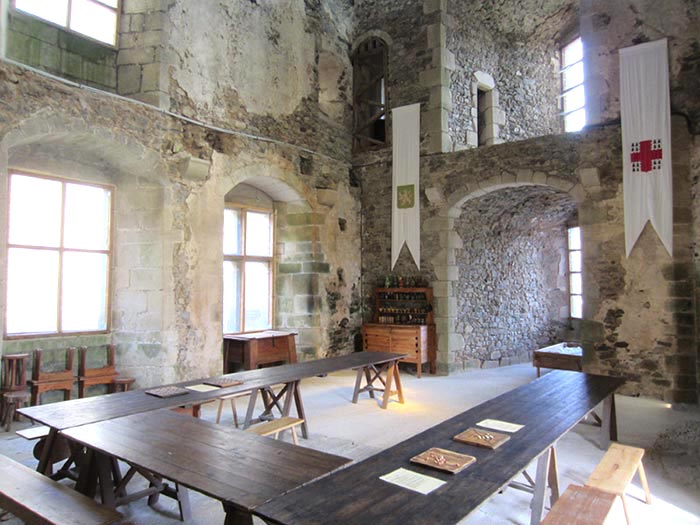The photograph captures the interior of an old, medieval stone castle with decaying stucco and exposed brick walls. The room features intricately detailed stonework and a vaulted ceiling, revealing a view of an upper level at a corner section. In the center, there are three low, round tables that evoke the imagery of a grand medieval round table, surrounded by benches of varying shades of brown—light and dark. The lighting suggests it is daytime, as rays of golden sunlight filter through the arched windows, casting a warm glow across the room.

Dominating the walls are two vertically hanging white banners. The banner on the right prominently displays a red cross, while the banner on the left features a green square with an emblem that seems to depict a lion-dragon hybrid. The stone walls behind these banners are constructed from round stones, meticulously held together at the corners by square bricks. The overall ambiance of the photograph is professional and meticulously captures the essence of a bygone era, rich with historical artifacts such as writing desks, chairs, and a cupboard, all devoid of any human presence.